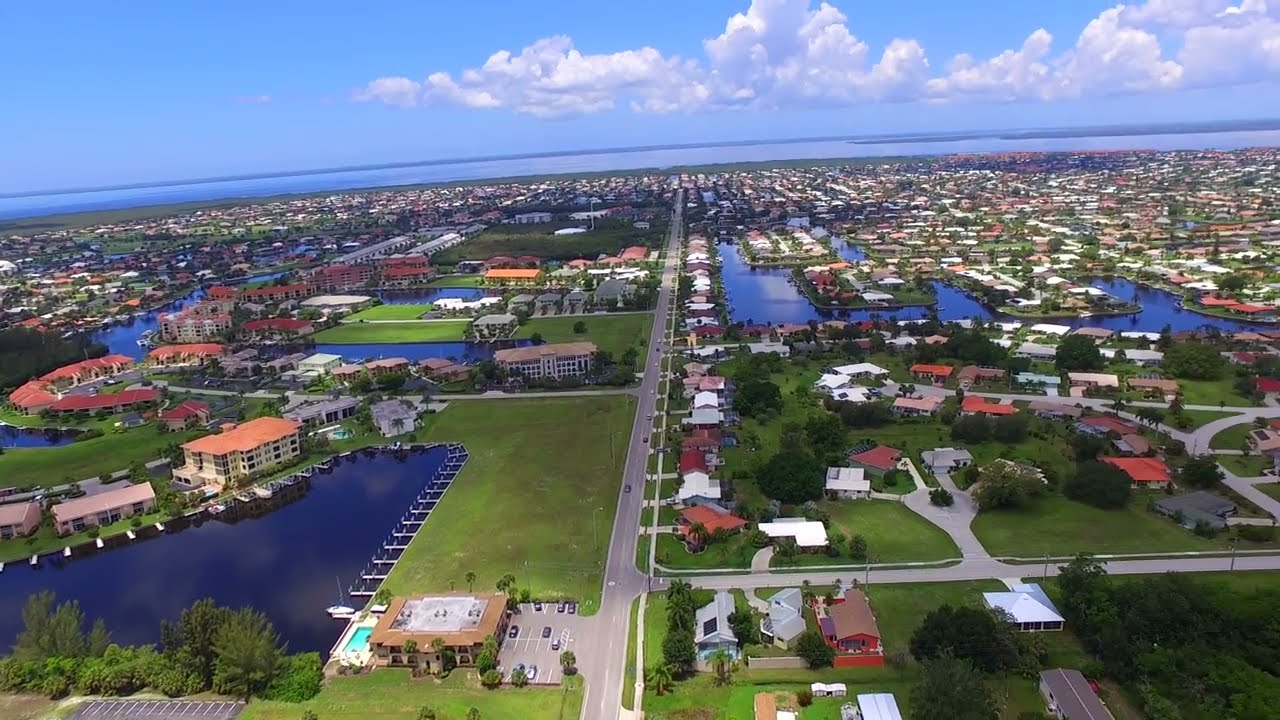An overhead, highly detailed aerial photograph in landscape orientation showcases a captivating coastal townscape at the edge of a massive body of water, either an ocean or a large lake, sprawling into the horizon. The photograph appears to be taken from a drone at a considerable height, providing a comprehensive view of the landscape below. On the right side of the image, two distinct, small, roundish islands are visible, each teeming with buildings adorned with orange or red tile roofs. These islands are encircled by water and are notably equipped with white docks that protrude into the surrounding river or lagoon. The foremost island features a prominent multi-story building, likely a hotel, along with several houses and a parking lot marked with white chalk or paint lines.

On the left side of the image, a dense forested area packed with vibrant green trees and bushes stretches out, potentially bisected by a thin creek or river. The contrasting landscape on the left forms a lush green buffer against the man-made structures on the right. In the background, towards the top half of the photograph, a sprawling expanse of clustered housing and assorted buildings peeks through, separated sporadically by patches of greenery. This residential area extends towards the horizon where the vast body of water meets the sky.

The sky itself is a serene light blue, dotted with soft, puffy white clouds, adding depth and a peaceful aura to the scene. The photograph embodies a realistic, representational style, capturing the intricate details and natural beauty of the coastal town and its surroundings from an elevated drone perspective.